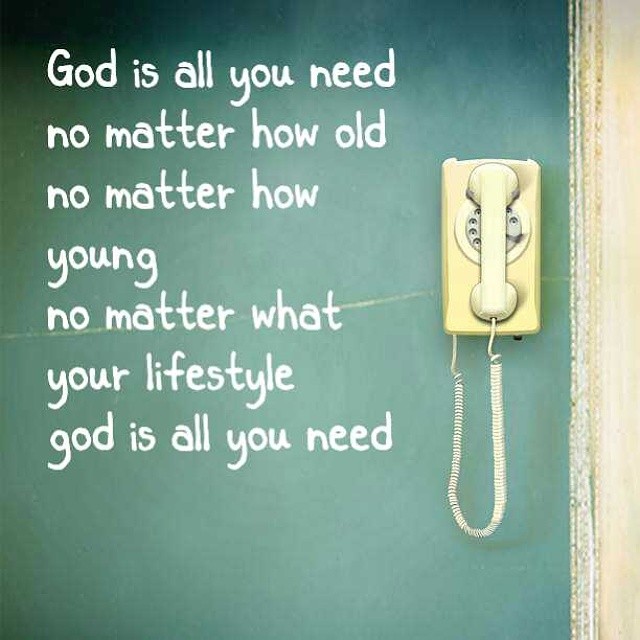The image depicts a motivational poster featuring a darkish green, school-style blackboard bordered by a very light-colored beige or white wood frame, especially noticeable on the right side. Mounted on the blackboard is a vintage, rectangular rotary telephone in a white or beige color, with its spiraling cord freely dangling below. The retro phone is positioned on the right side of the blackboard. On the left side of the blackboard, written in a casual white font, is the inspirational message: "God is all you need, no matter how old, no matter how young, no matter what your lifestyle, God is all you need." The repetition of the phrase "God is all you need" emphasizes its message, though the lowercase 'g' in the concluding line adds a subtle variance.